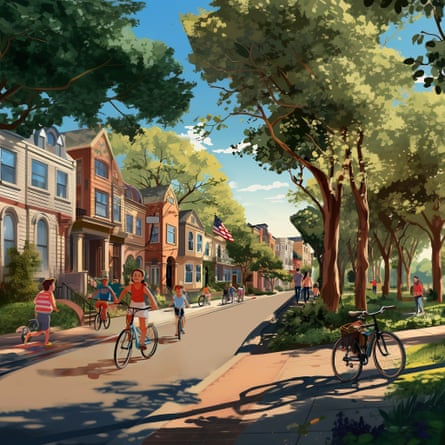The image is a realistic, computer-generated illustration of an idealized American downtown neighborhood scene. Dominated by soft earth tones and beiges, the setting exudes a vibrant, community-oriented atmosphere on a sunny summer day. On the left side, a row of townhomes closely nestled together is shaded by large, lush trees. An American flag waves prominently from one of the homes, evoking a sense of patriotism. The right side features a small path leading to a park bustling with activity, including children playing and adults relaxing. The street, tapering from the lower left corner to the center, is devoid of cars, emphasizing pedestrian and bicycle traffic. A girl in a red tank top and white skirt rides a blue bike with a basket, followed by a boy on another bike, while other kids run and play with their dogs. The clear blue sky dotted with a few clouds enhances the idyllic, almost nostalgic charm of the scene.